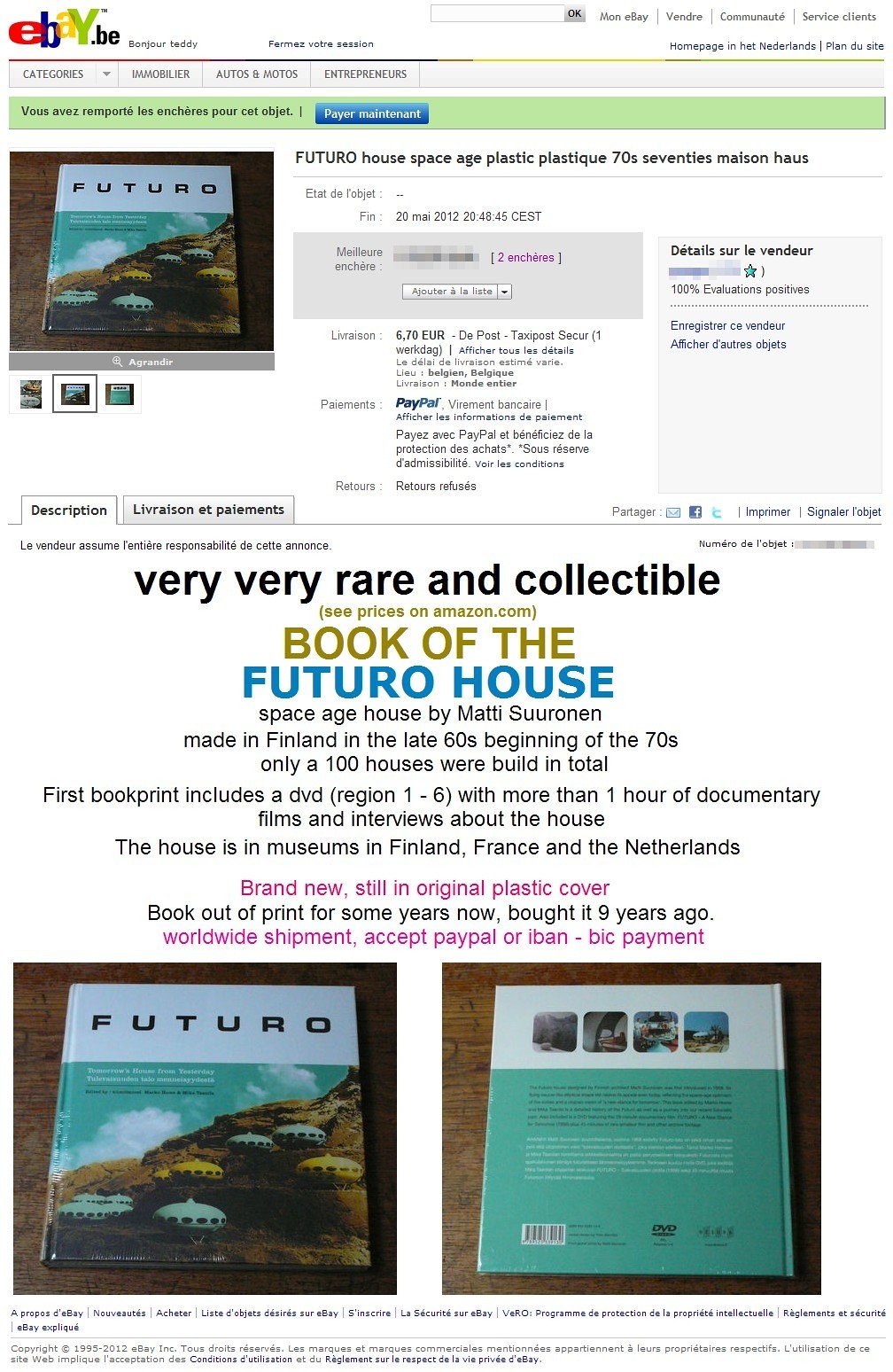This image is a tall, rectangular screenshot of an eBay listing. In the upper left corner, the colorful eBay logo is prominently displayed with the 'E' in red, 'B' in blue, 'A' in yellow, and 'Y' in green alongside the '.be' suffix in black. Directly beneath the logo is a photograph of a book titled "Futuro." The adjacent text on a white background reads "Futuro House Space Age Plastic Plastique Seventies Maison House," followed by paragraphs written in French. Positioned towards the bottom are more photographs of the book, likely showing both its cover and back.

Highlighted text above the additional pictures proclaims the book as "very, very rare and collectible" in black font. Just below, a green text encourages viewers to "see prices on Amazon.com," and immediately underneath in blue font, it says "Futuro House."

Details regarding the book reveal that it covers the Futuro House, a space-age dwelling designed by Matti Suuronen in Finland during the late 60s and early 70s, with only 100 units built. The initial print of the book includes a DVD (region 1 through 6) featuring over an hour of documentary films and interviews about the house. These unique houses are also noted to be in museums located in Finland, France, and the Netherlands. The entire screenshot displays a colorful blend of white, red, blue, yellow, green, gray, purple, and pink, typical of eBay's user interface showcasing categories and auctions.